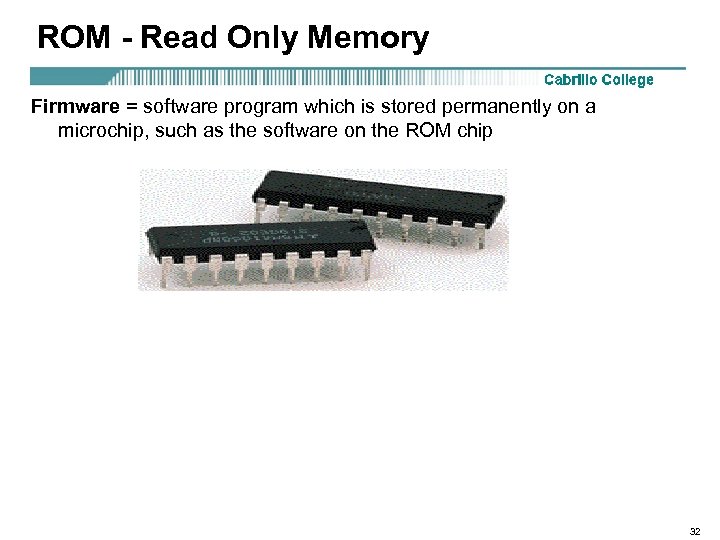The image appears to be an educational slide from a computer class, likely associated with Cabrillo College, featuring a white background with a headline that reads "ROM, Read-Only Memory." Below the headline, there is a decorative horizontal border. The left segment of the border is solid blue, transitioning to vertical blue lines that fade to white towards the right, with the text "Cabrillo College" positioned at the far right end of the border. 

Underneath the border, there is explanatory text in black lettering: "Firmware = Software Program which is stored permanently on a microchip, such as the software on the ROM chip." A black and white photograph follows the text, showing two microchips, presumably ROM chips. These rectangular black chips have hard-to-read white letters and numbers on their surfaces. They also feature 10 visible pins on their bottom sides, projecting shadows and appearing somewhat grainy and blurry in the image.